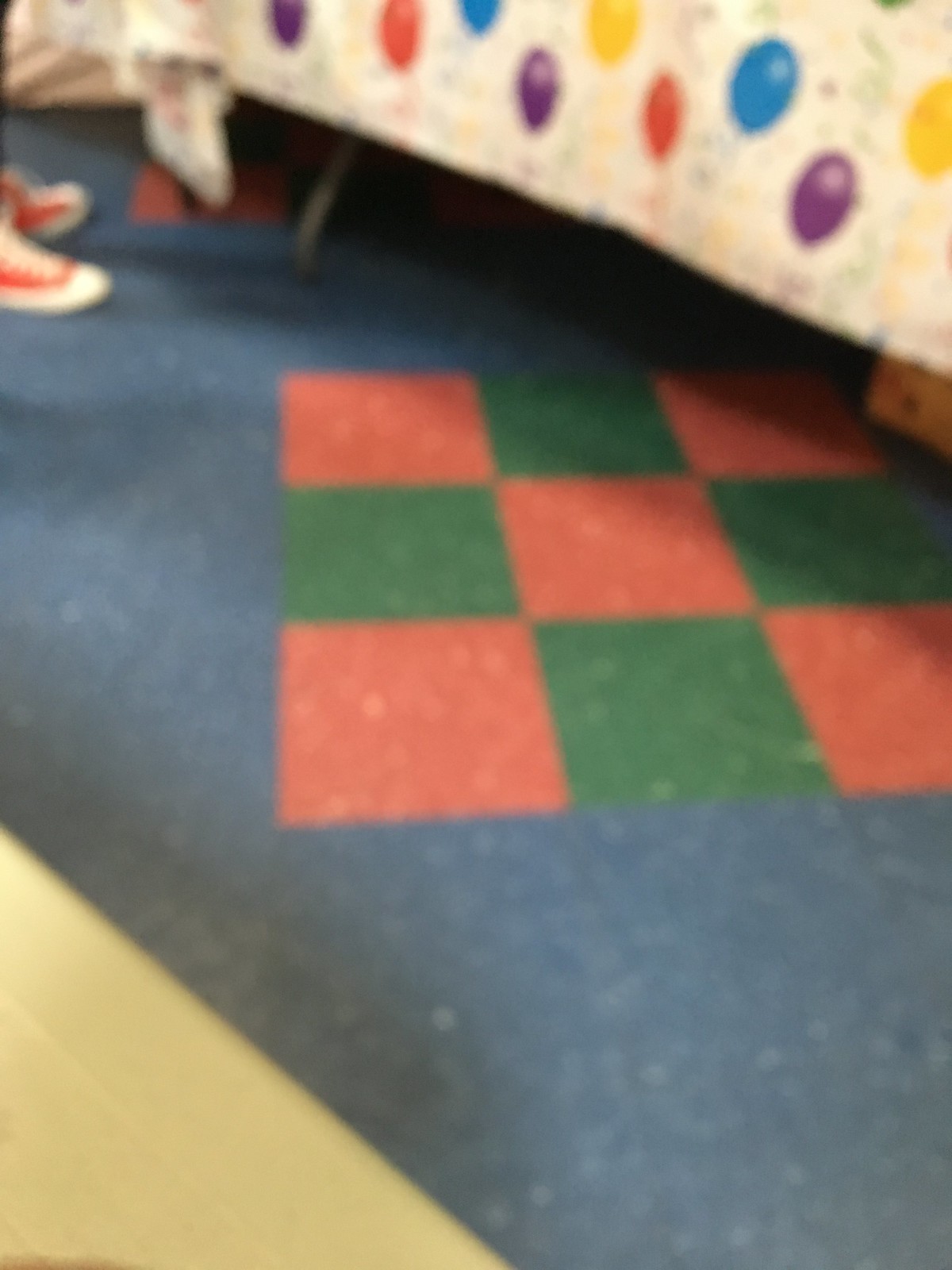The photograph is slightly out of focus, capturing the corner of a child’s room. Central to the image is the lower portion of a child's bed, characterized by a whitish bedspread adorned with a vibrant, multi-colored balloon pattern, creating a joyous and playful atmosphere. The bed appears welcoming and cheerful against the backdrop. Lying beneath the bed is a predominantly blue rug featuring a prominent design: a large, three-foot by three-foot checkerboard pattern with alternating orange and green squares, adding a dynamic touch to the room's decor. Partially visible is another similar checkerboard section, hinting at the rug's extensive design. The flooring around the rug is a light blonde wood, providing a warm contrast to the blue and patterned elements. In the upper right corner of the image, a pair of red tennis shoes casually lies on the floor, adding a pop of color and a hint of everyday life to the scene.